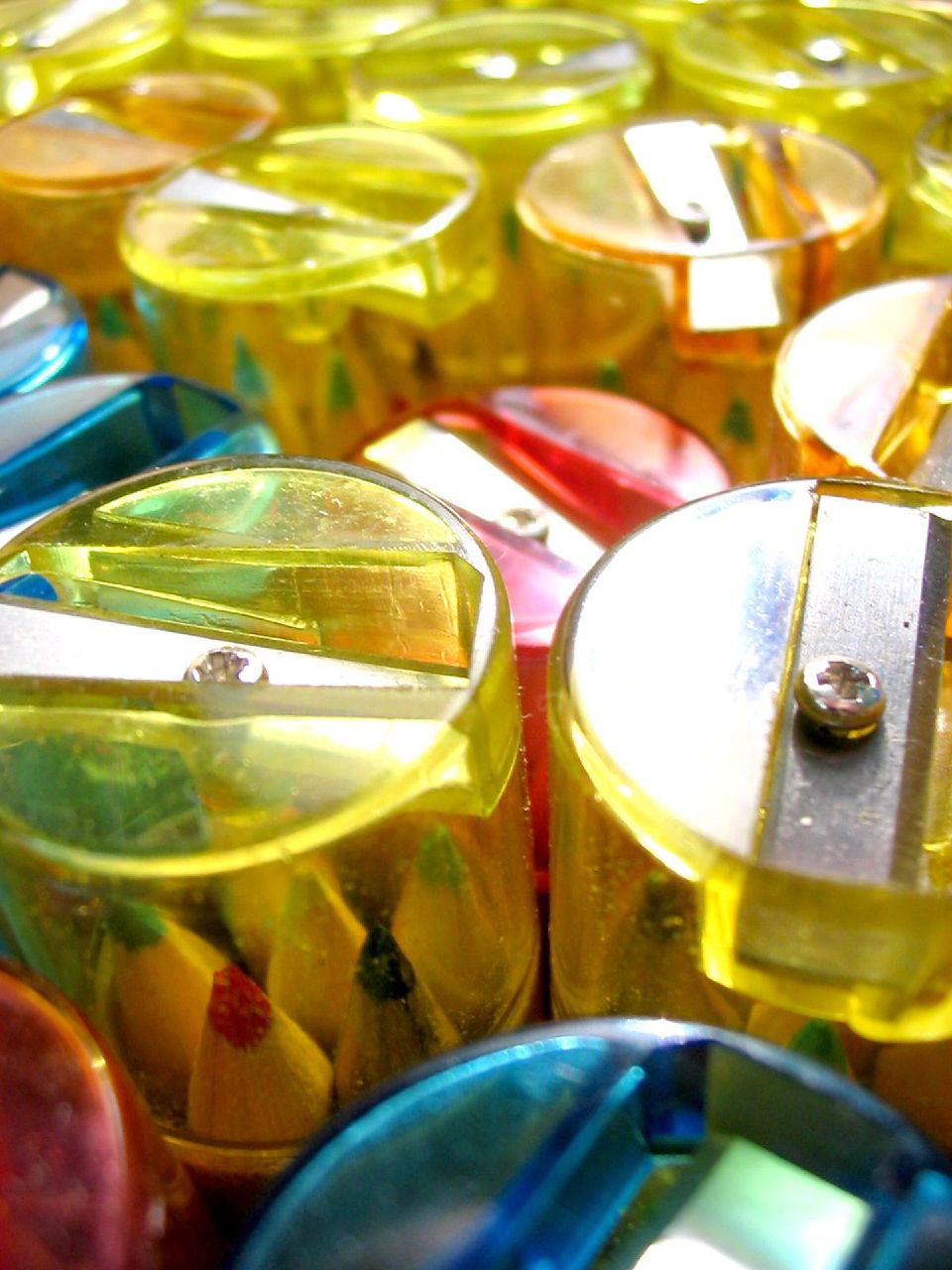This is a digital photograph of several cylindrical pencil containers, each made from clear plastic and featuring colored pencils with fairly hard lead designed for artists' drawing. The pencil containers are capped with amber or colored plastic lids that have built-in silver pencil sharpeners at the top. The sharpeners are secured with a small Phillips head screw in the center. In the image, you can see a range of pencil colors, including red, green, yellow, blue, orange, and possibly brown, with neatly sharpened tan tips visible. The containers vary in color – predominantly blue, red, and yellow – and are organized in rows, with some appearing in the foreground and others slightly out of focus in the background. Each container's translucent design allows the colors of the pencils inside to be easily seen.